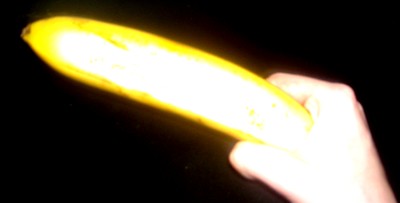In a photograph set against a stark black background, a person's hand is prominently displayed, grasping a ripe, unpeeled banana. The hand, visible from the wrist to the fingers, firmly holds the fruit at its base with a clenched fist. The banana, bathed in ample light, reveals its vibrant yellow hue, indicating its peak ripeness, while the smooth texture of the peel reflects the illumination. The composition of the image highlights the readiness of the person to enjoy the banana, capturing the moment of anticipation. The focused lighting accentuates both the contours of the banana and the detailed features of the hand, creating a striking visual contrast against the dark backdrop.